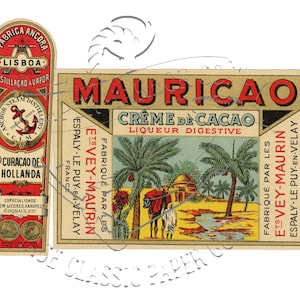In this image, on a light beige or cream-colored background, there are two distinct posters side by side. The poster on the right is rectangular with red, black, and light blue text that reads "Morikau Kremdi Kakao Liquor Digestive." The text "Maracau" is prominently displayed in red letters with black outlining. Below this text is an intricate drawing depicting an outdoor ground area filled with yellow sand, where a couple of people are walking amidst trees, with a small hut-like building in the backdrop. There are also text and possible import stamps on the left and right sides of the drawing. The background of this poster provides an aesthetic complement to the vivid colors of the text.

To the left side of this poster, there is another long, thin poster with a semicircular top, featuring a red background. The text on this poster includes "Fabrica Ancora Lisboa," although it's partially cut off on the left side, and below this is a logo with an anchor, followed by the words "Caraco of Dihalenda." This poster stands taller than the one on the right, creating a varied visual composition. There is a watermark in the middle of the entire image, but it is not very clearly visible and does not detract from the detailed content of the posters.